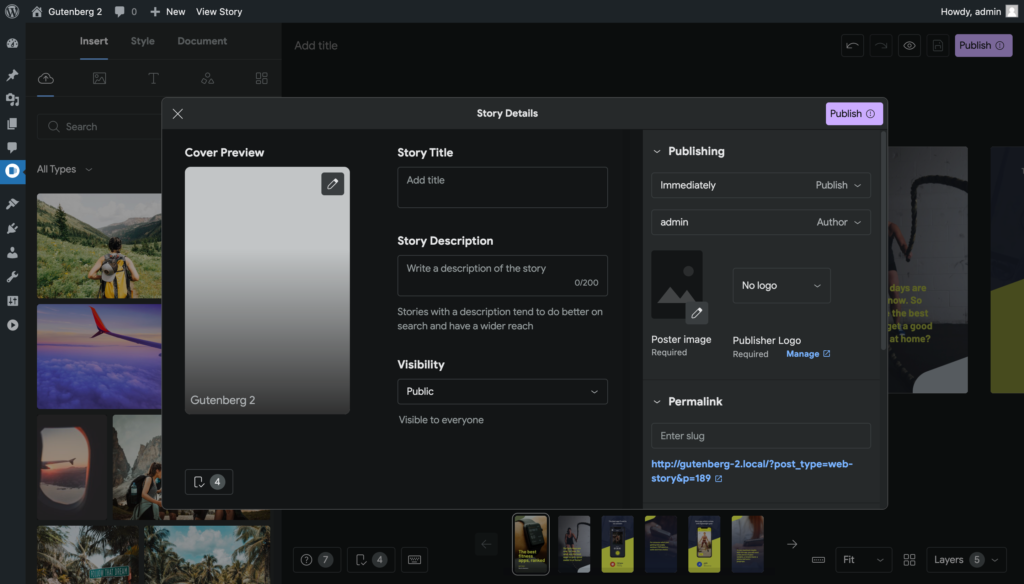Here is a cleaned-up and detailed caption for your image:

---

The screenshot showcases a web interface with a predominantly black background. The top left corner features a white "W" enclosed in a circle, followed by a home icon, indicating navigation elements. The page is titled "Gutenberg 2." In the top right corner, the interface greets the user with "Howdy Admin."

On the left-hand column, there is a vertical arrangement of photographs. The top image depicts a person standing outdoors amidst rolling hills and mountains. Below it, a photo captures the tail of an airplane soaring above the clouds. The third image down in the column shows a woman wearing a backpack, situated in an outdoor setting. The final and largest image in this column presents a street scene with a focus on a street sign and palm trees in the background.

Adjacent to this column, to the right, the text reads "Cover Preview," with a large gray rectangle resembling the shape of a smartphone screen. In the top right of this section, a black square contains an image of a pencil, probably indicating an edit function.

In the lower left corner of the screenshot, the text "Gutenberg 2" is repeated. To the right, a section labeled "Story Details" provides fields for "Story Title," "Ad Title," and "Story Description." An accompanying text box prompts the user to "Write a Description of the Story," noting that "Stories with a description tend to do better on search and have a wider reach." 

Further down, a visibility option states "Visibility: Public, Visible to Everyone." On the far right column, prominently displayed, there is a "Publish" button, ready for the user to finalize their story.